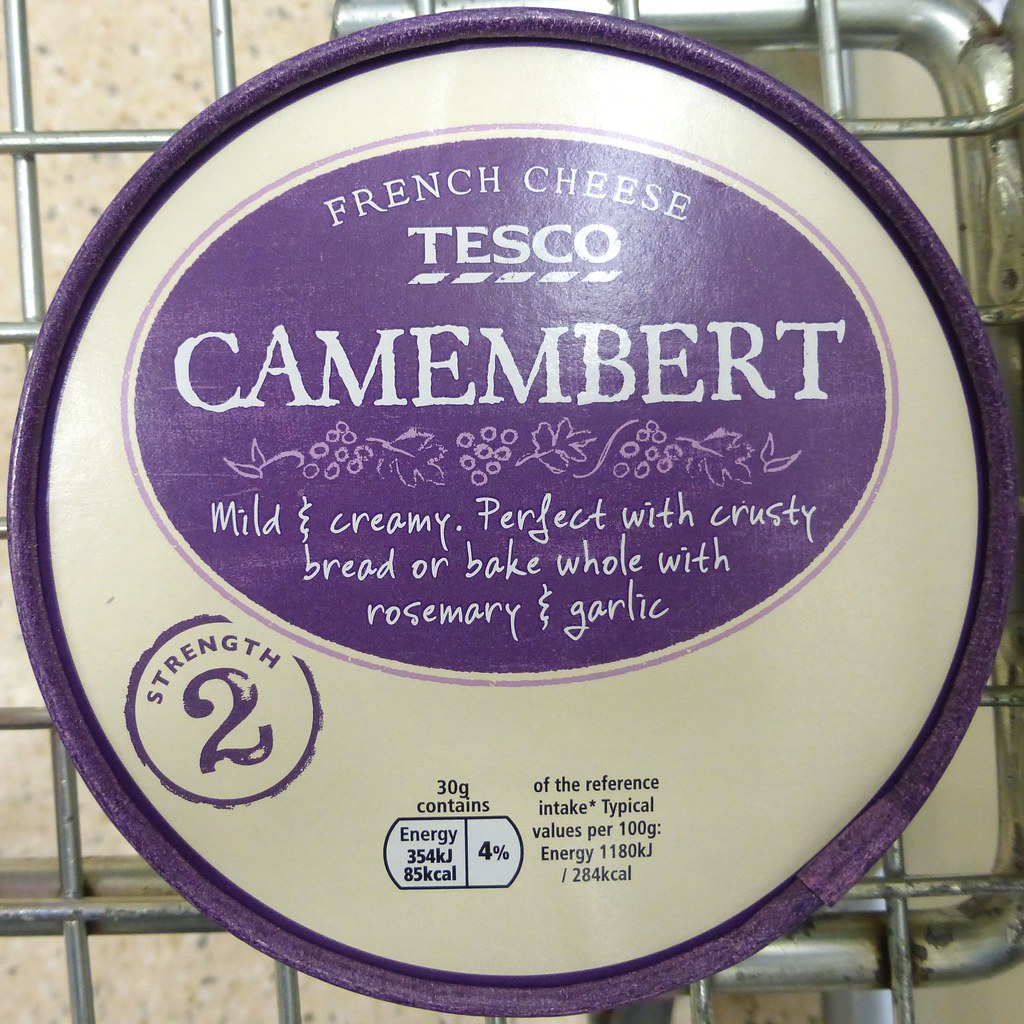This image features the lid of a food product, specifically Camembert cheese by Tesco. The circular lid has a prominent purple border and a large horizontal oval in the center that occupies about two-thirds of the lid. Inside the oval, white text states "French Cheese," followed by "Tesco" and "Camembert." Below this, smaller white text reads, "Mild and creamy, perfect with crusty bread or bake whole with rosemary and garlic." Surrounding this text are subtle designs of grapes and leaves. In the lower-left corner of the lid, there is a smaller circle with a purple border that indicates "Strength 2." In the lower center, black text details the nutritional information: "30g contains, Energy 354 KJ, 85 Kcal, 4%," followed by "of the reference intake, typical values per 100g, Energy 1180 KJ, 284 Kcal." The background of the lid gives the impression of a metal grating.